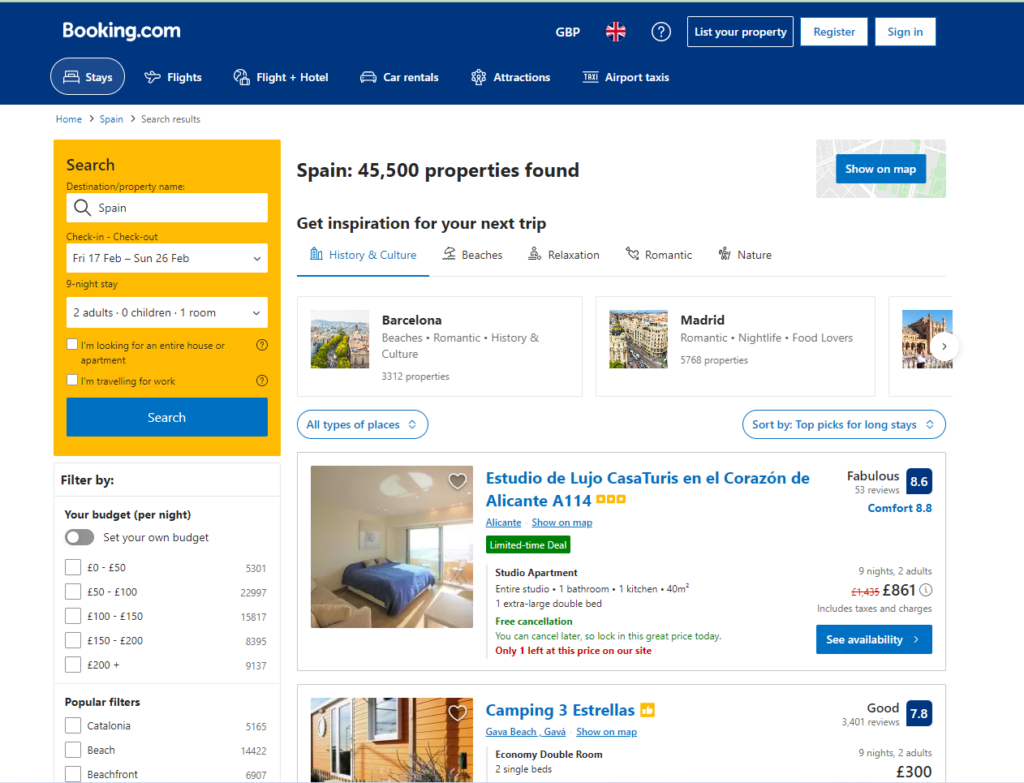The image depicts the top section of a website, specifically booking.com. The layout is slightly wider than it is tall, with a predominantly square aspect ratio. 

At the very top, there is a dark blue banner that occupies approximately 10-15% of the image's height. The banner features white text and icons. In the upper left corner, the booking.com logo is prominently displayed. 

Beneath the banner is a horizontal navigation bar composed of white, horizontally-aligned ovals representing different categories: 
- The first one, labeled "Stays," is highlighted and features an icon of a bed. 
- The second, "Flights," is marked with a plane icon. 
- The third combines a house icon and the label "Flight and Hotel."
- The fourth shows a car icon and the text "Car Rentals."
- The fifth includes a light bulb icon and is labeled "Attractions."
- The sixth oval displays a taxi icon accompanied by the text "Airport Taxis."

In the upper right corner, there are various elements:
- "GBP" followed by the British flag indicating the currency.
- A white circle with a question mark inside, serving as a help or info icon.
Additionally, there are buttons labeled:
- "List your property"
- "Register"
- "Sign in"

The left-hand side of the image contains filters, presumably for refining search results, while various listings are shown on the right side.